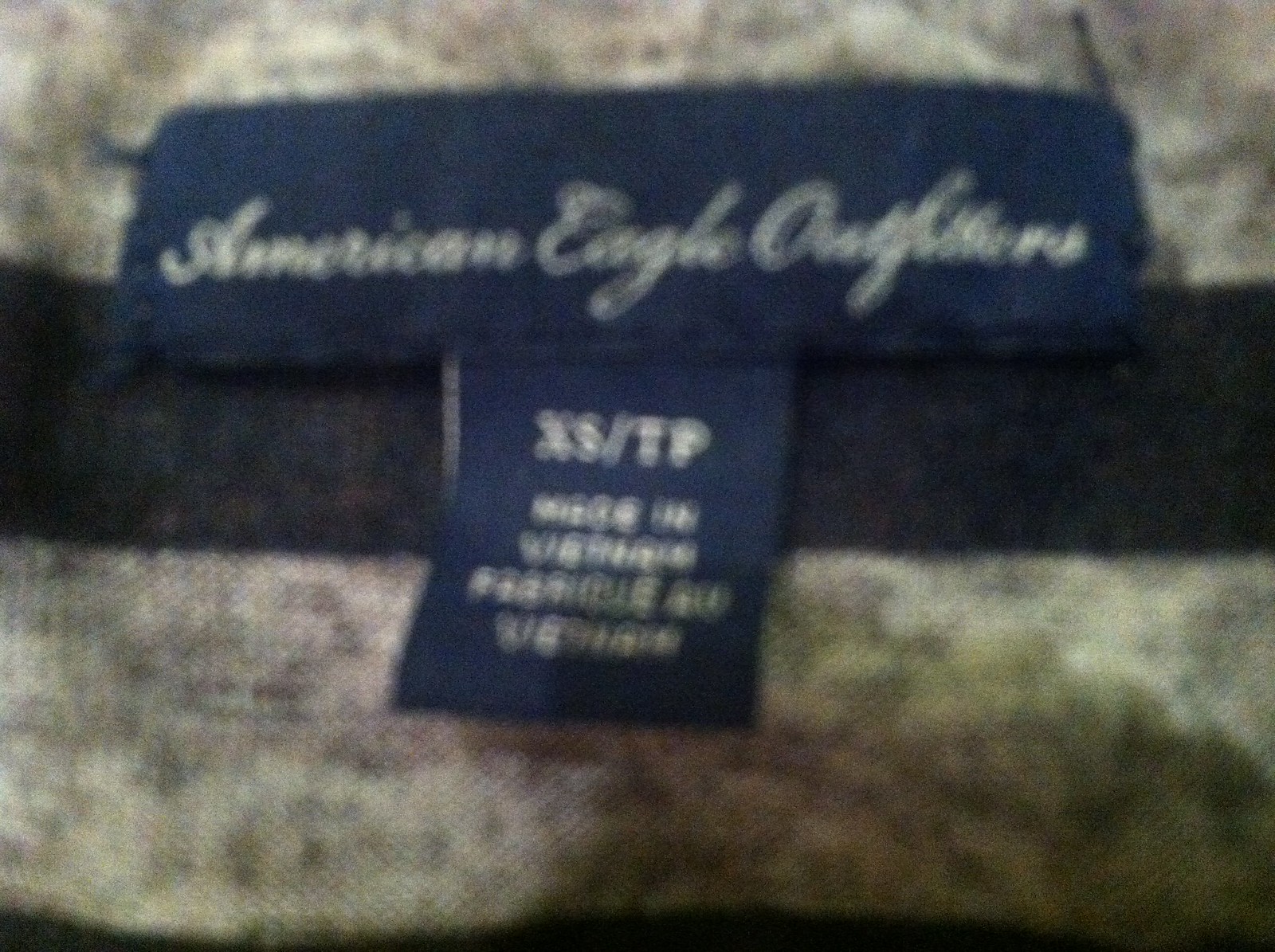This close-up photograph features a piece of gray clothing with black dots and stripes implying pigmentation and pattern variation. Central to the image is a tag from American Eagle Outfitters, though the image is quite blurry. The prominent tag includes a large dark blue rectangle with white cursive text reading "American Eagle Outfitters," and overlapping this tag is a smaller square tag indicating size "XL" (extra small) alongside "TP." There is an inscription beneath it stating "Made in Vietnam," along with additional Spanish text that is difficult to discern due to the blurriness. The background of the clothing appears to be a mix of gray and black with black stripes and dotting, possibly indicating that the item is a gray and black striped sweater.